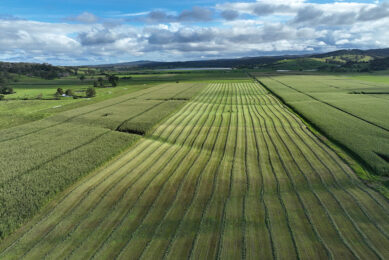The image depicts a vast, well-maintained agricultural field extending into the horizon. The field is characterized by its vibrant green hue, with neat, straight rows of crops running through the middle, possibly grapevines or similar tall crops, tilled and meticulously arranged. On either side of these rows, the grass appears to be taller and slightly overgrown. The photograph is taken from a high vantage point, providing a panoramic view that includes distant rolling hills or small mountains blanketed in trees, with occasional clearings of open grass. The scene is complemented by a partly cloudy sky with grayish-white clouds scattered across a bright blue expanse. In the far distance to the left, you can spot sparse trees and possibly a lake, adding to the tranquility of the landscape. The entire composition exudes a serene, pastoral beauty, capturing the essence of rural farmland.